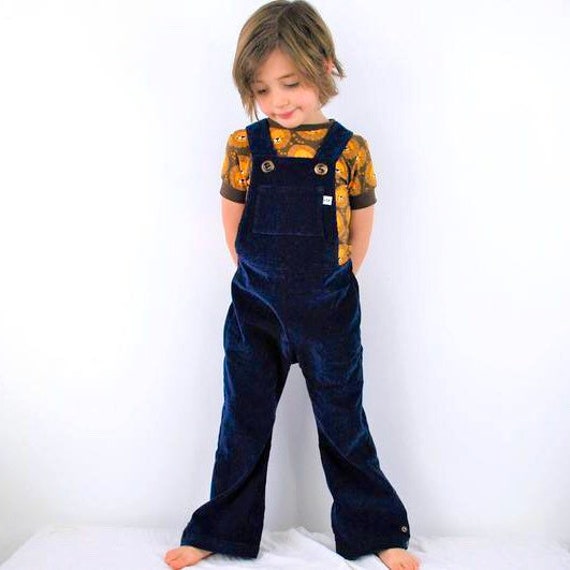This photograph captures a young boy, likely around the age of three to five years old, standing barefoot on a tabletop draped with a white cloth. The boy has longish, dirty brown hair and is clad in dark blue, corduroy overalls with flared legs, secured by gold buttons—one of which bears an "S." He wears a shirt underneath featuring a yellow and orange circular design with a greenish collar. The backdrop is stark white, emphasizing the child's downward gaze and subtle smile. His hands are positioned behind his back, and he stands with his legs slightly spread. The overall scene conveys a mix of innocence and curiosity as the child appears to contemplate something with a gentle, introspective expression.